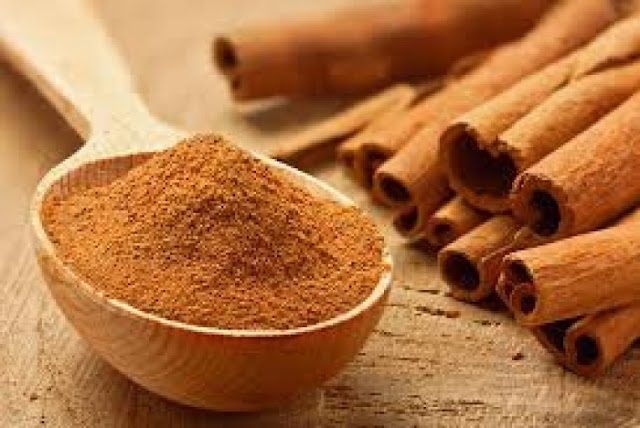This color image is a close-up of a distinctive wooden spoon on a wooden tabletop. The spoon, possibly handmade or expensive, features visible wood grain and is filled with a heaping pile of light brown, finely ground cinnamon powder. Its handle starts in the upper left corner and extends towards the center of the frame but is partially cut off, emphasizing the close-up perspective. To the right of the spoon, there is a neat stack of cinnamon sticks—approximately 12 or 13 in total, arranged in two layers. The bottom layer consists of around seven sticks, while the upper layer has about three partially visible sticks. The rich, golden-brown hue of the powder and the natural texture of both the wooden spoon and the cinnamon sticks highlight the rustic and tactile nature of the scene.